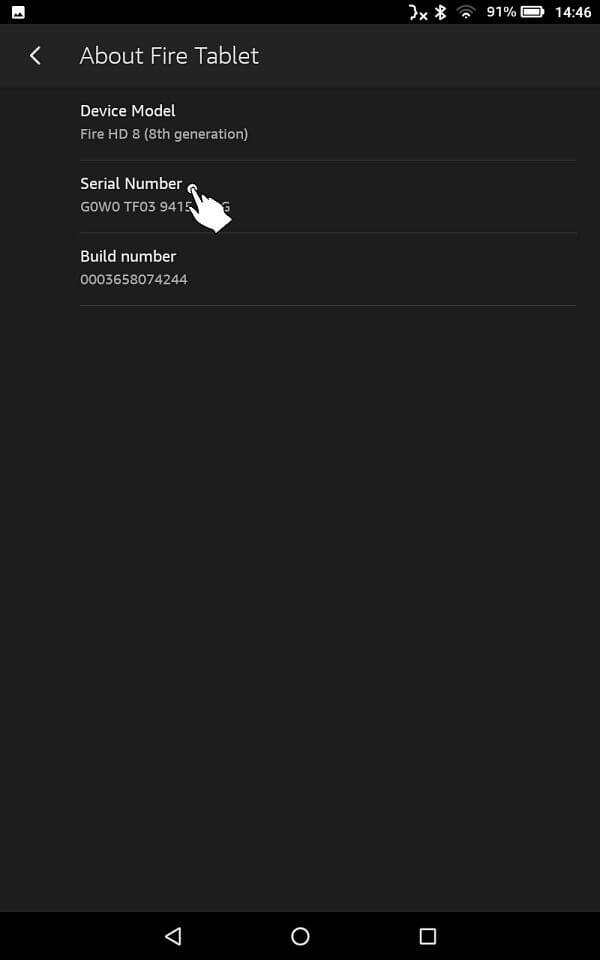This screenshot depicts an Android mobile app displayed in portrait mode. The screen has a rectangular shape, and the icons are neatly arranged. 

- **Top Bar Information**:
  - Top-left corner: A small white square icon representing an attachment or image feature.
  - Top-right corner: A series of icons indicating the phone’s status.
    - A silhouette of a person with a white "X" in front of their mouth suggests the phone is on silent mode.
    - The Bluetooth icon is illuminated in white, indicating it is activated.
    - The Wi-Fi signal is shown at two out of four bars.
    - The battery percentage is at 91%.
    - The current time is displayed as 14:46 (2:46 PM).

- **Main Content**:
  - A header reads "About Fire Tablet," rendered in white font against a lighter gray background. This header includes a back button positioned to the left.
  - Below the header, details about the tablet are displayed:
    - **Device Model**: Fire HD 8 (8th Generation).
    - **Serial Number**: The beginning of the serial number "G0W0 TF03 9415" is visible, but the last part is obscured by a pointing hand cursor, revealing only the final letter "G".
    - **Build Number**: 0003658074244.